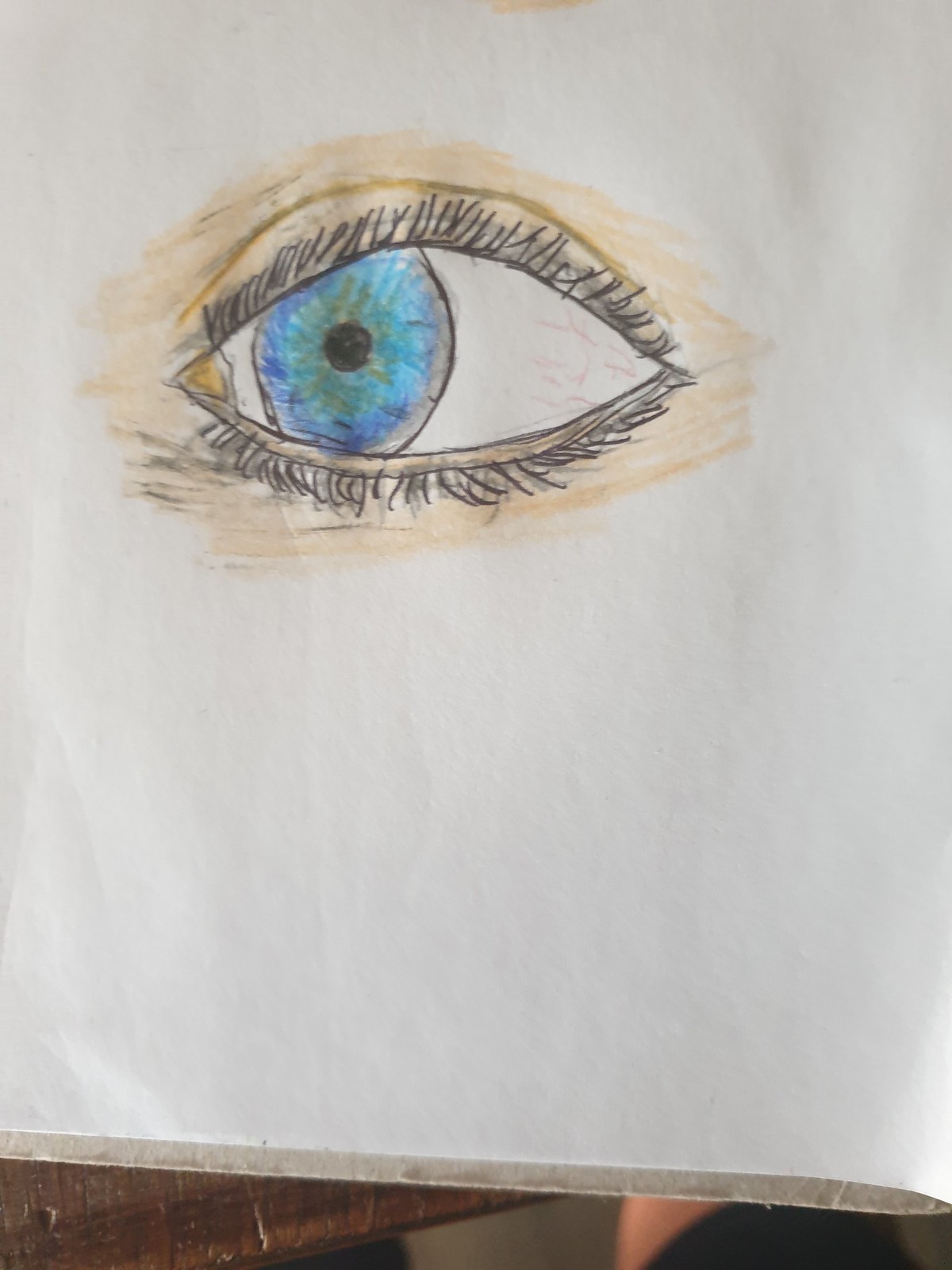A close-up view of a beautifully detailed eye is captured, showcasing an intricate makeup application. Surrounding the striking blue eye is a shimmering bronze eyeshadow, creating a vibrant contrast against the eye's natural color. The top eyelid features a dark glaze, adding depth and drama. Wispy, dry lashes adorn the upper and lower lids, with the lower set being more prominently visible. Delicate white and red veins run across the white of the eye, adding a realistic touch. The eye, predominantly blue, intriguingly has a subtle green tint encircling the pupil. In the background, a subtly folded piece of white paper adds texture to the composition, though it remains mostly out of focus.